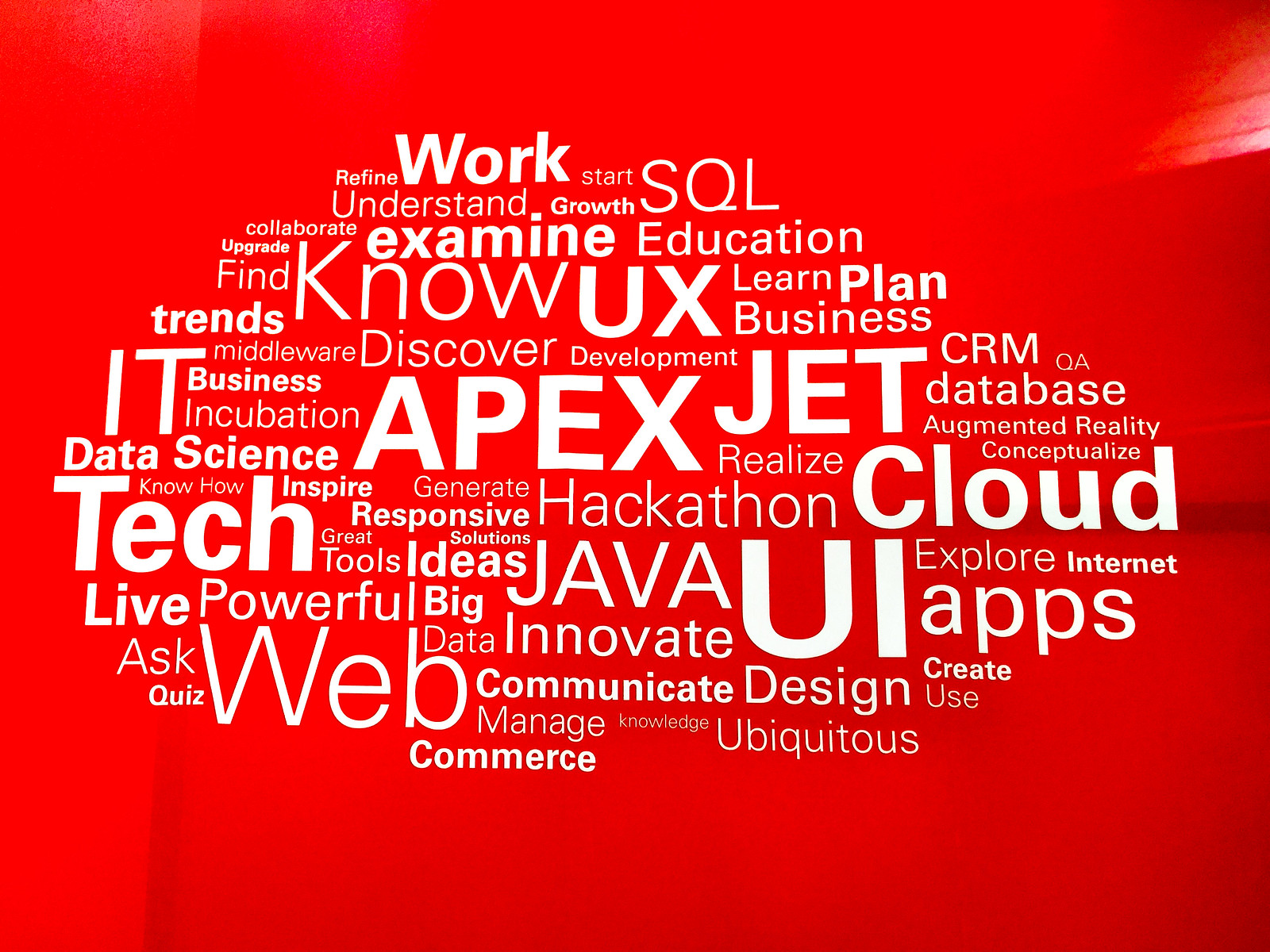The image is a wide rectangular word cloud set against a bright red background, with subtle shading in the top right corner, center right, and bottom left corner. The word cloud, which has an almond-like shape wider than it is tall, with a slight upward tilt on the left side, features white text in various fonts and sizes. Prominent words such as “UI,” “apex,” “cloud,” “UX,” “jet,” and “tech” stand out clearly. Other notable terms include "SQL," "collaborate," "examine," "upgrade," "growth," "find," "know," "business," "development," "augmented reality," "conceptualize," "CRM," "QA," "database," "middleware," "discover," and "realize." Smaller words like "refine," "work," "start," "understand," "education," "plan," "IT," "incubation," "trends," "learn," "tech," "web," "apps," "knowledge," "Java," "solutions," and "great" are also visible, each contributing to the technology-centric theme of the design.